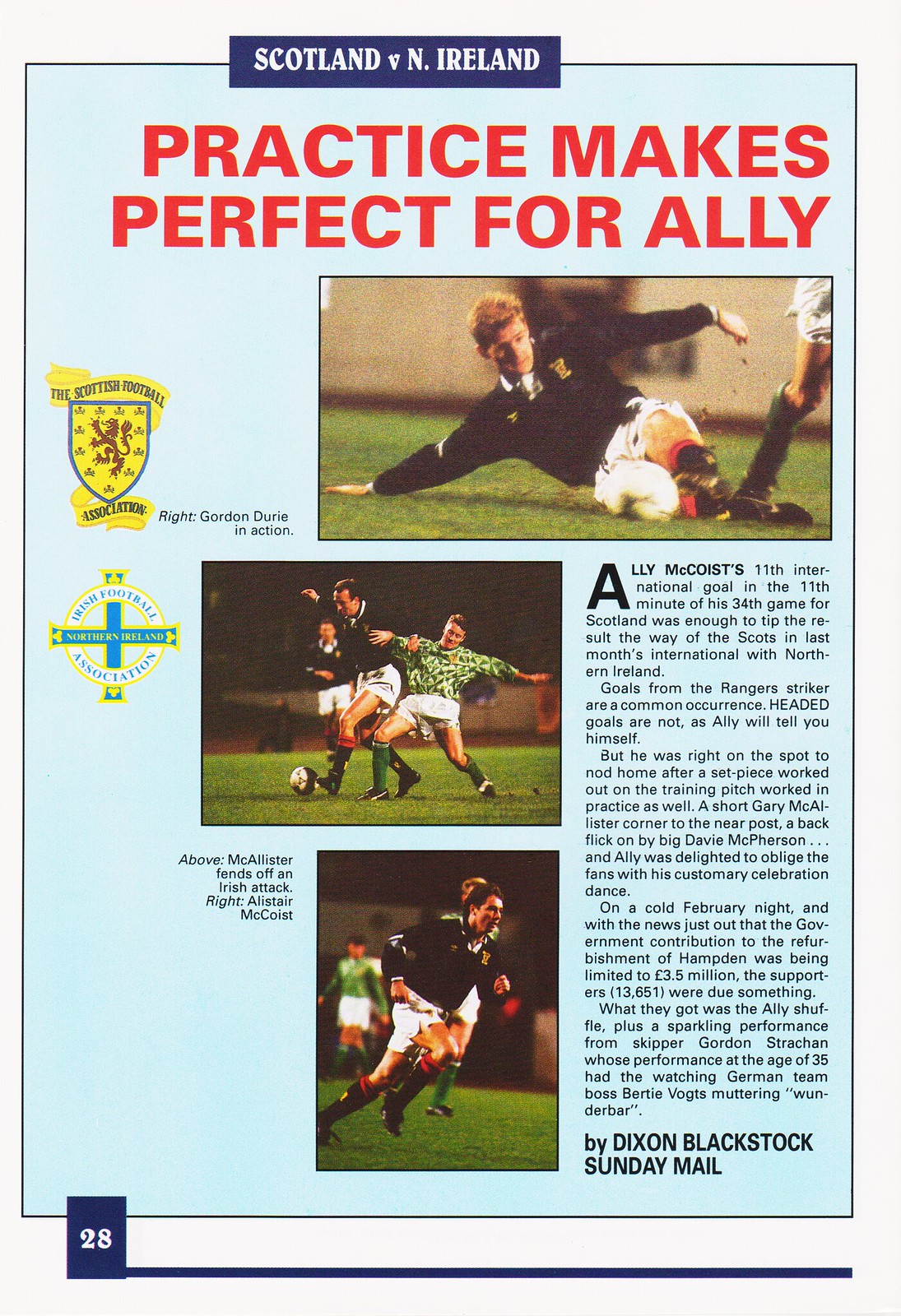This image appears to be a newspaper cover or flyer for an upcoming soccer match between Scotland and Northern Ireland. The vertically aligned, rectangular page features a prominent headline at the top in white all-caps letters against a blue rectangular background, announcing "SCOTLAND VERSUS NORTHERN IRELAND." Below this, in striking red all-caps letters, is the article title, "PRACTICE MAKES PERFECT FOR ALLY."

The layout includes a thin blue border encompassing the entire page. Adjacent to the headline, two emblems appear: one featuring a shield with a lion and the other a cross. The article includes three color photos showcasing soccer action. The first image captures a man in a dark jersey and white shorts kicking a ball while on the ground. The second photo shows three players, all in white shorts, vying for the ball. The third image, located at the bottom, depicts a man running on the field, though no ball is visible in this photo.

To the right of the photos is a text block comprising a few paragraphs in dark blue font, which discuss the practice and details related to the match. The page concludes with a byline reading "Dixon Blackstock, Sunday Mail." Additionally, there are short captions off to the left of two of the photos, identifying the individuals featured in them.